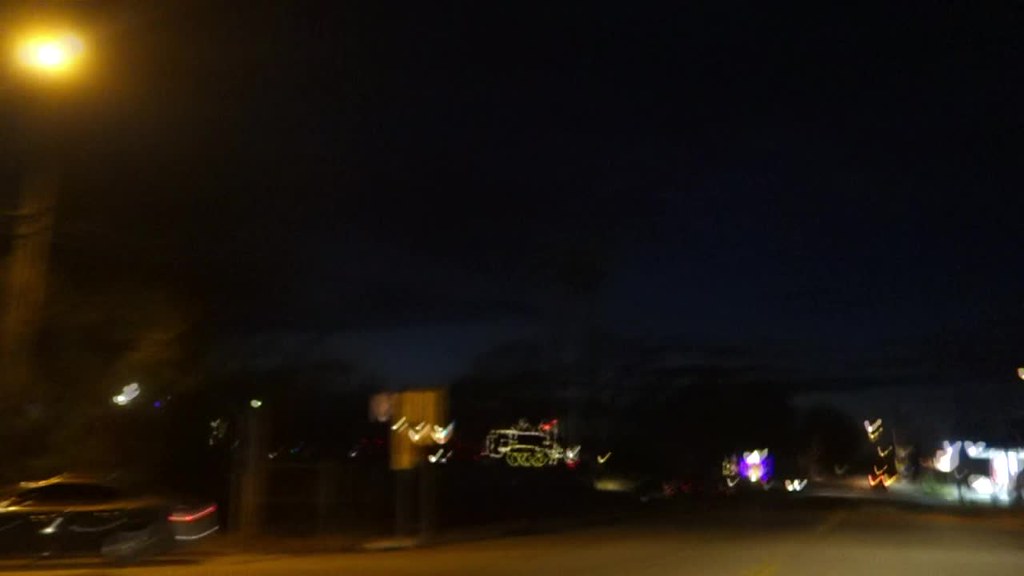The photograph, taken at night, captures a blurry yet bustling street scene. At the center of the image is a restaurant adorned with a navy blue canopy over its entrance. The establishment is illuminated by a mix of fluorescent neon lights and attached building lights, creating a vibrant glow. In the foreground, a road is visible, with the blurred motion of passing cars, their lights streaking through the frame. A black sedan is discernible at the cross street, adding to the dynamic atmosphere. Above, a tall tree stretches into the sky, with a bright light at its peak shining down onto the street below. In the distant background, the lights of other businesses line the road, contributing to the lively nighttime ambiance.